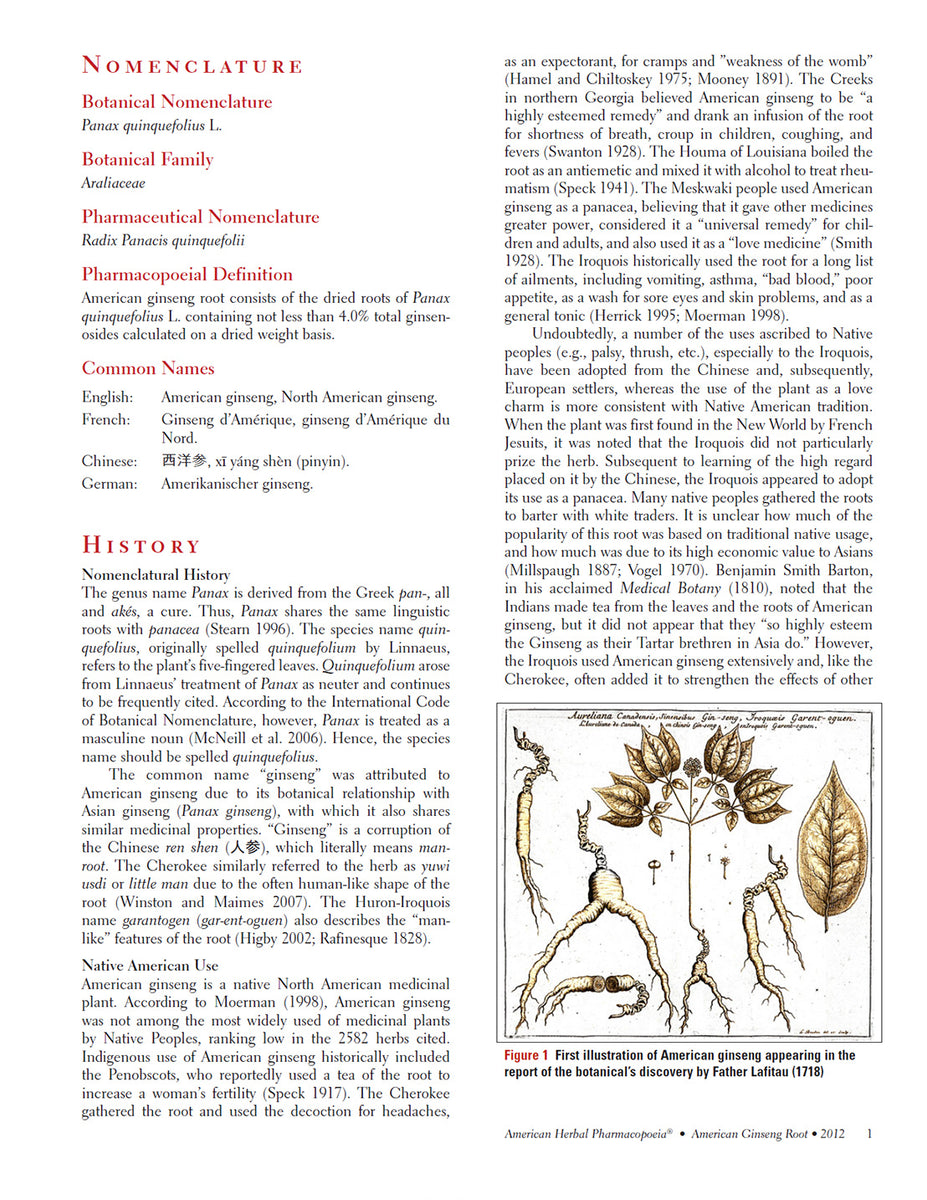The image depicts a page from a printed material, formatted into two columns. At the top left corner, the headline "Nomenclature" is highlighted in red, followed by the subheading "Botanical Nomenclature." Underneath, the text in black reads "Panax crinifolius L," and then in red again "Botanical Family," specified as "Aureliacea" in black text. The left column continues with detailed information, including headers such as "Pharmaceutical Nomenclature," "Pharmaceutical Definition," and "Common Names." 

A section titled "History" in red provides an etymological explanation of the genus name "Panax," derived from the Greek "pan" (all) and "akēs" (cure), sharing roots with the word "Panacea" (Stern, 1996). The column finishes with three paragraphs of detailed historical context.

The right column contains two long paragraphs of additional information. Towards the bottom, there is a rectangular area outlined with thin black lines containing illustrations of leaves and roots in a brown hue. Under these images, labelled "Figure 1," the caption notes this as the "first illustration of American ginseng, appearing in the report of the botanical's discovery by Father [name], 1718." The entire layout intricately combines taxonomy, historical context, and visual elements to provide a comprehensive presentation of the botanical subject.